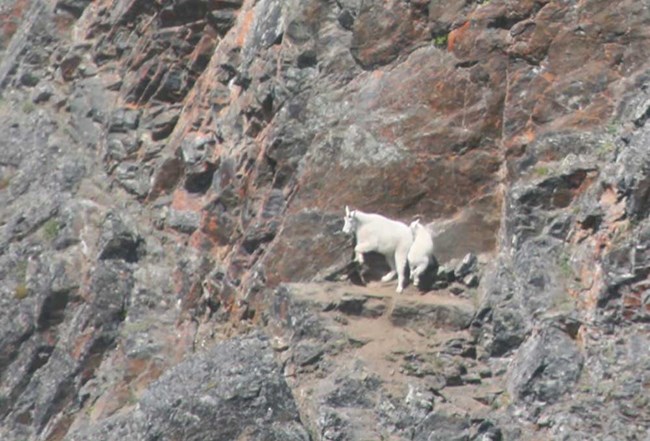This image depicts a low-quality photograph of a mountainous landscape, characterized by rugged and rocky terrain, primarily in dark gray with streaks of reddish ore, likely iron. The mountain, dotted with sparse vegetation in the indentations of the rock, features a steep cliff face inclined at approximately 70 to 80 degrees. Two white goats can be seen in the middle of the picture, positioned on a narrow outcrop covered with patches of brown dirt. The leading goat, facing away from the camera, has horns, while the second goat trails closely behind, oriented sideways. They appear poised to traverse a more precarious section of the cliff. The photograph makes it evident that the path forward is daunting, as the only visible egress is back towards the foreground to the right, along a dirt path interspersed within the rocky surroundings.